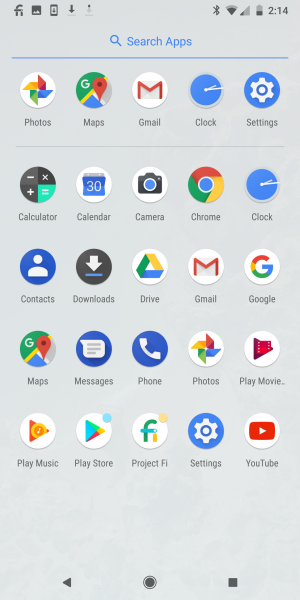A vertical image captured from a smart device screen. The background is a medium gray with minimal texture or dimension, appearing fairly flat. At the bottom, there is a slight hint of dimension and subtle color merging, but it's not very prominent.

In the upper left-hand corner, there are various clickable icons displayed in black. On the upper right-hand corner, icons indicate the device’s status, including Bluetooth connectivity, signal strength, battery life, and the current time, which reads 2:14.

Below these indicators, there's a search bar with the text "Search apps" accompanied by a magnifying glass icon, underlined with a blue line. The main screen displays an array of app icons arranged in a grid, each represented by a circular image with the app name written in black beneath it.

Here are the apps in order from top to bottom:

- Top row: Photos, Maps, Gmail, Clock, Settings
- Second row: Calculator, Calendar, Camera, Chrome, Clock
- Third row: Contacts, Downloads, Drive, Gmail, Google
- Fourth row: Maps, Messages, Phone, Photos, Play Movies
- Fifth row: Play Music, Play Store, Project Fi, Settings, YouTube

At the very bottom of the screen, there are navigation buttons: a triangle pointing left (Back button), a circle (Home button), and a square (Recent Apps button).